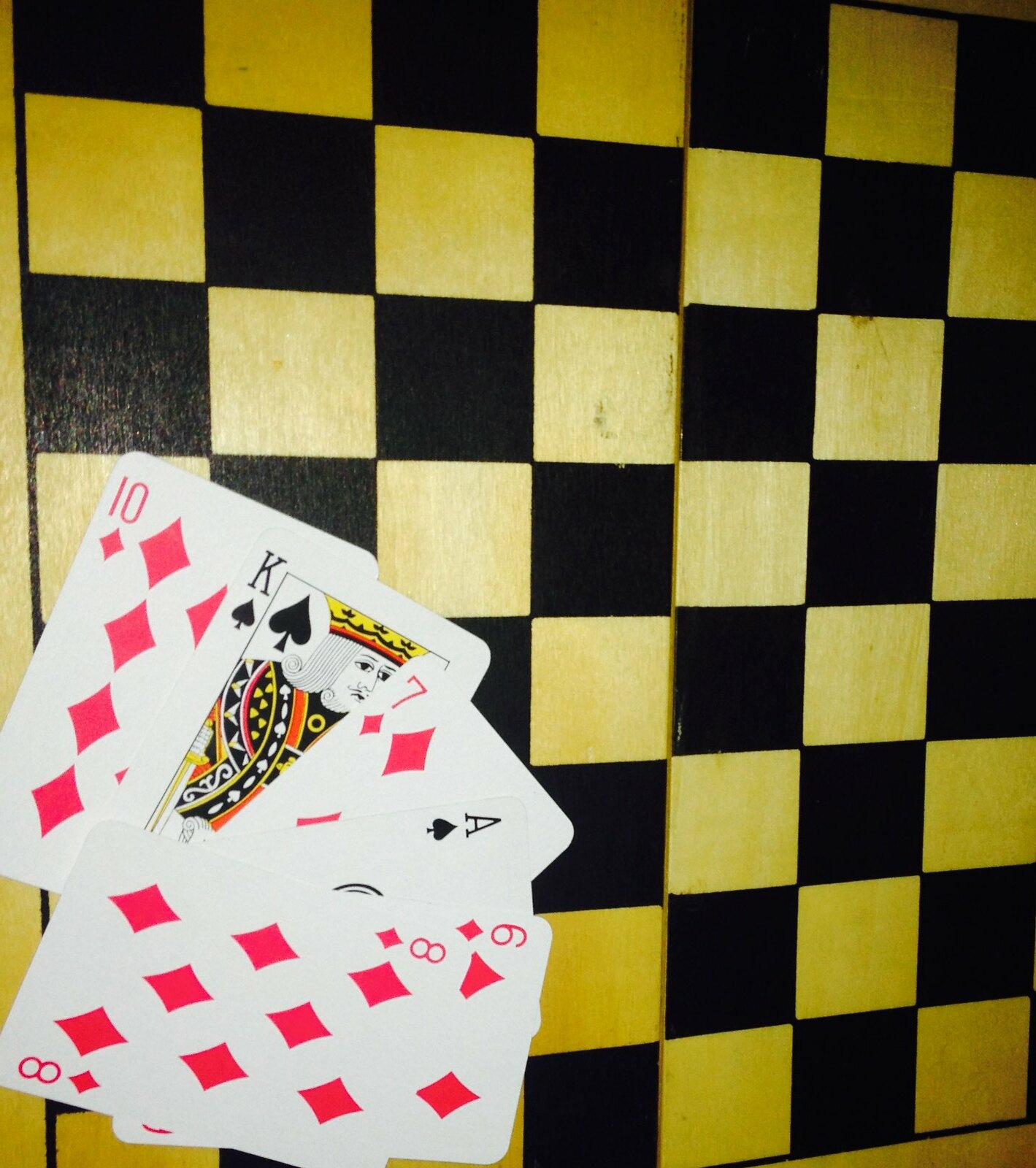The image depicts a top-down view of a checkers table, showcasing a game board with a black printed checkers pattern on a light tan, almost yellowish wood surface. Dominating the bottom left quadrant of the frame is a fanned-out arrangement of six standard playing cards, forming a semi-circular arc from bottom to top in a clockwise direction. The cards, which partially overlap, are as follows: a King of Spades, a Seven of Diamonds, an Ace of Spades, a Six of Diamonds, and an Eight of Diamonds. Each card has a classic white background with traditional markings; red icons and numbers for the diamonds and black for the spades. The King card features a typical depiction of a king, illustrated in black and white with detailed pen-like strokes. His crown is adorned in yellow with various symbols, and his royal attire is highlighted with accents of yellow and red. The overall composition presents a blend of strategic games, merging the worlds of checkers and card play in a single engaging image.